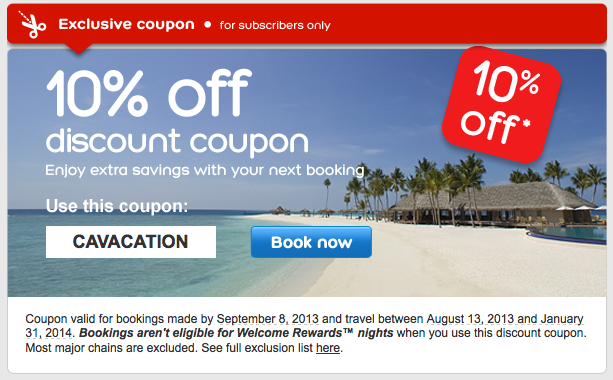The image features a prominent promotional graphic with several distinct elements. At the top, there is a large red square containing a white illustration of scissors cutting a dashed line, accompanied by the text "Exclusive Coupon" and a small white circle labeled "For Subscribers Only." The background is primarily blue, with a gradient effect creating a lighter blue halo around the edges. The main visual attraction is a picturesque beach scene showcasing clear blue water, pristine white sand, a quaint pavilion, and lush green palm trees.

Superimposed on this idyllic backdrop is bold white text reading "10% Off Discount Coupon" followed by smaller text stating "Enjoy extra savings with your next booking. Use this coupon." Below this, there is a white square with black text that says "Cave Vacation," and a blue button with white lettering that says "Book Now."

In the upper right corner of the image, another red box announces "10% Off" with a small asterisk next to it. At the bottom of the image, a white box contains detailed terms and conditions in black text, stating: "Coupon valid for bookings made by September 8, 2013 and travel between August 13, 2013, and January 31, 2014. Bookings aren't eligible for Welcome Rewards nights when you use this discount coupon. Most major chains are excluded. See full exclusion list here," with the word "here" underlined.